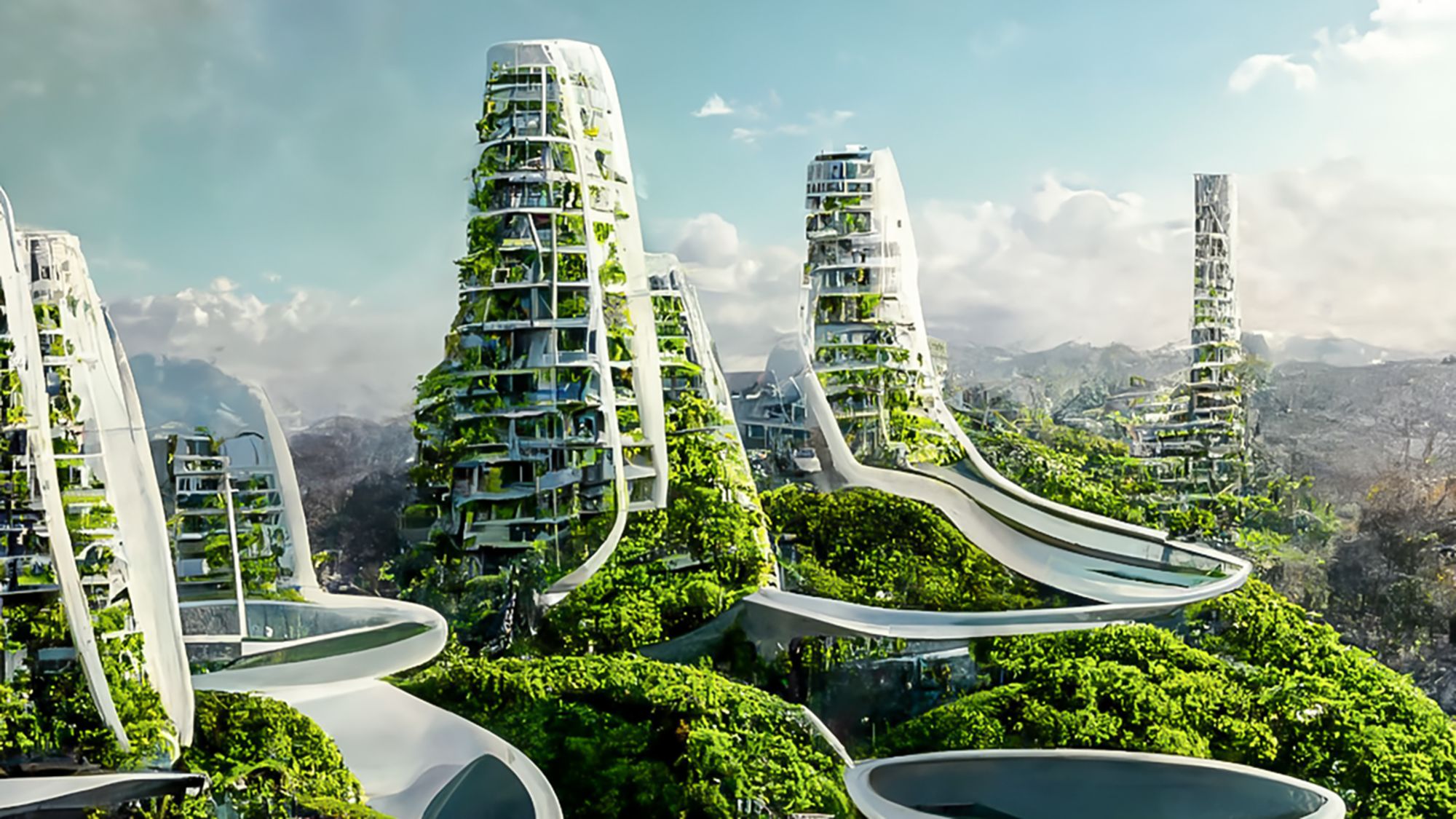This is a highly detailed digital rendering of a futuristic cityscape, reminiscent of a science fiction setting with a slight Aztec architectural influence. The image features four to five extraordinarily tall, white cylindrical structures that gradually taper at the top, making them somewhat pyramid-like but closer to cylinders. These unique buildings are entirely enveloped in lush greenery, with trees and plants growing up their sides, merging architecture with nature. Positioned among verdant mountains blanketed with dense trees, these towering edifices are interconnected by fantastical, slide-like white paths or roads, some of which lead to large, enigmatic dark ovals that could be pools or other structures. The sky above is a gray-blue hue, adorned with prominent white clouds, enhancing the sense of height and grandeur of the buildings. The overall scene is a mesmerizing blend of advanced urbanism and abundant organic growth, suggesting a harmonious coexistence of futuristic design and natural elements.